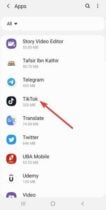This is an extremely blurry screenshot resembling a phone interface, specifically within the apps section. The top one inch of the image features a light blue background. On the left side, there's a black "greater than" sign pointing left, accompanied by the word "apps" to its right. On the right side of this top bar, three vertical dots are followed by a search icon. Below this, a white search bar appears, containing the word "All" on the left side, a number "3" beside it in thin light-blue text, and a white background extending downward until the bottom inch which is light blue again.

Running down the left side of the screenshot, nine icons are faintly visible, each corresponding to an app. To the right of these icons, bolded black text identifies each app, with smaller black text underneath that is illegible due to the blurriness. Notably, the fourth app icon has a red, thick, bold arrow pointing to it, angled down to the right, and approximately two inches long. The app being highlighted by the arrow is "TikTok."

At the bottom center of the screenshot, three dark gray vertical lines are visible with a dark gray circle containing a lighter gray center situated in the middle. The right side of the bottom features another dark gray circle, but its contents are not discernible.